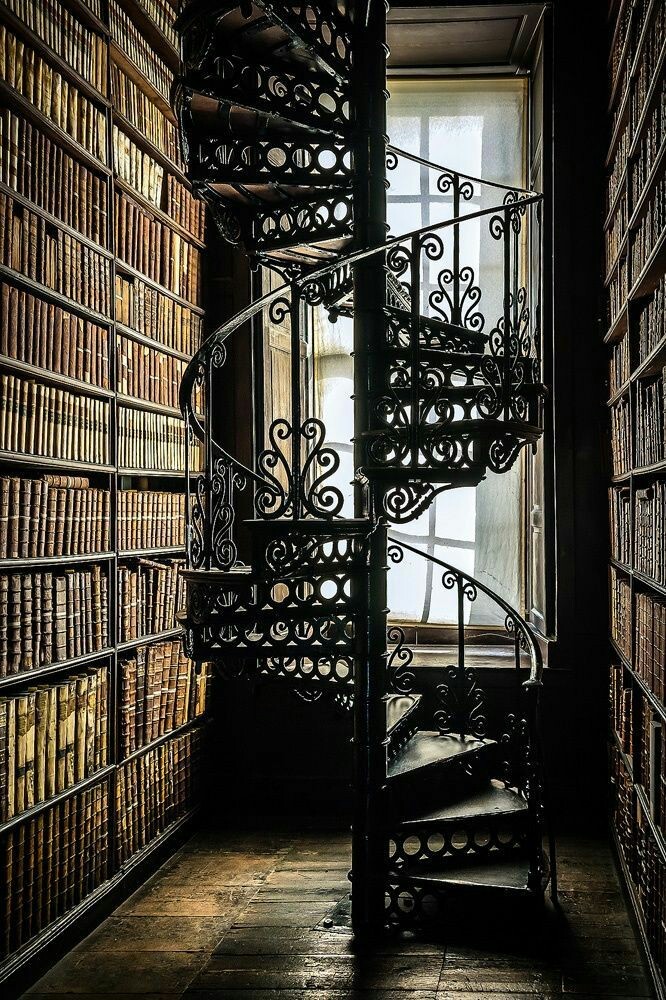This image depicts a narrow, dimly-lit room with an ornate, black metal spiral staircase at its center, stretching upwards through the frame. The staircase, reminiscent of an intricate cylindrical structure, provides access to towering bookshelves on both sides, filled with tightly-packed, aged books in tans and browns. The floor is a beautiful brick-patterned hardwood, enhancing the rustic charm of the space. A large, paned window sits at the back, extending from about a foot and a half above the floor to near the ceiling, allowing a soft, natural light to faintly illuminate the room. The overall ambiance is one of a secluded, vintage library, accentuated by the winding staircase and the towering rows of bookshelves that stretch up to approximately 10 to 12 feet high.